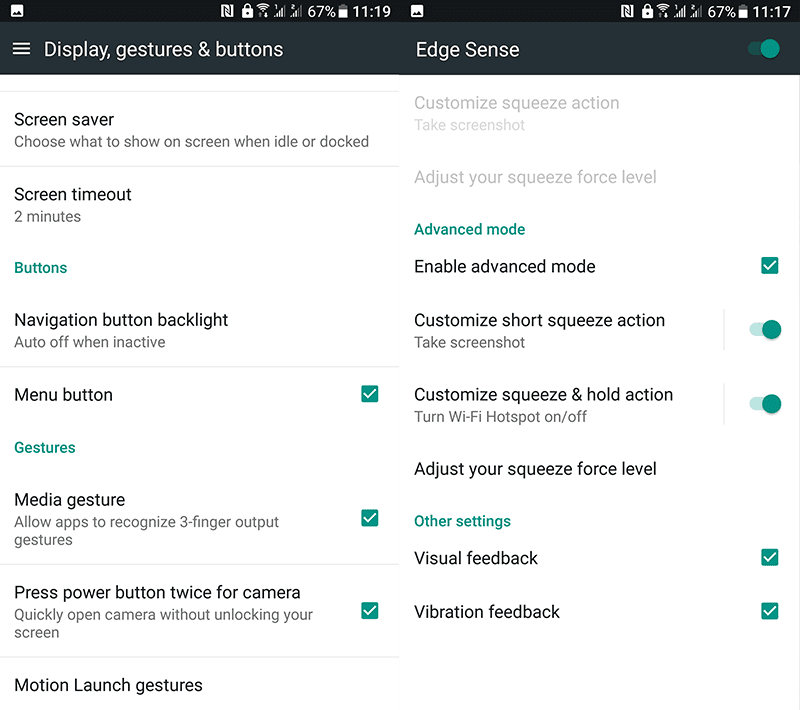This image features two HTC smartphone screenshots displayed side by side, showcasing the distinct EdgeSense functionality and various gesture controls available on the device.

On the left screenshot, the title "Display, gestures & buttons" is prominently displayed at the top in large white font against a black header, with a menu icon to its left. The screen has been scrolled down to reveal a white background divided by a gray line right under the header. Below this, "Screen saver" is highlighted in large black font, followed by the description "Choose what to show on screen when idle or docked" in smaller black font. The next line introduces the "Screen timeout" button in light blue font, and beneath this are additional sections titled "Navigation button backlight," "Menu button," and "Gestures," each dealing with specific functionalities related to screen and button interactions. The 'Gestures' section is in bold blue font, followed by subcategories including "Media gesture" and "Press power button twice for camera." Further down, the section "Motion Launch gestures" is visible.

On the right screenshot, the title "EdgeSense" is displayed at the top left, indicating the exclusive feature available on HTC U11 or U12 models. Below the header, the screen exhibits customized settings for the squeeze functionality labeled as "Customize squeeze action" and "Adjust your squeeze force level," both of which are grayed out. The section "Advanced Mode" is prominently displayed in bold blue font beneath these options. Subcategories under "Advanced Mode" include "Enable advanced mode," "Customize short squeeze action," and "Take a screenshot," with a toggle switch, which is turned on, to the right. Further down, "Customized squeeze and hold action" leads into "Turn Wi-Fi hotspot on/off," featuring another active toggle switch. Under these settings, "Adjust your squeeze force level" is listed again, followed by the "Other settings" category. This final category displays checked boxes for "Visual feedback" and "Vibration feedback."

The detailed side-by-side display of the screenshots provides a comprehensive view of the customizable touch and squeeze features available on this HTC smartphone model, catering to users who seek to personalize their device interactions.